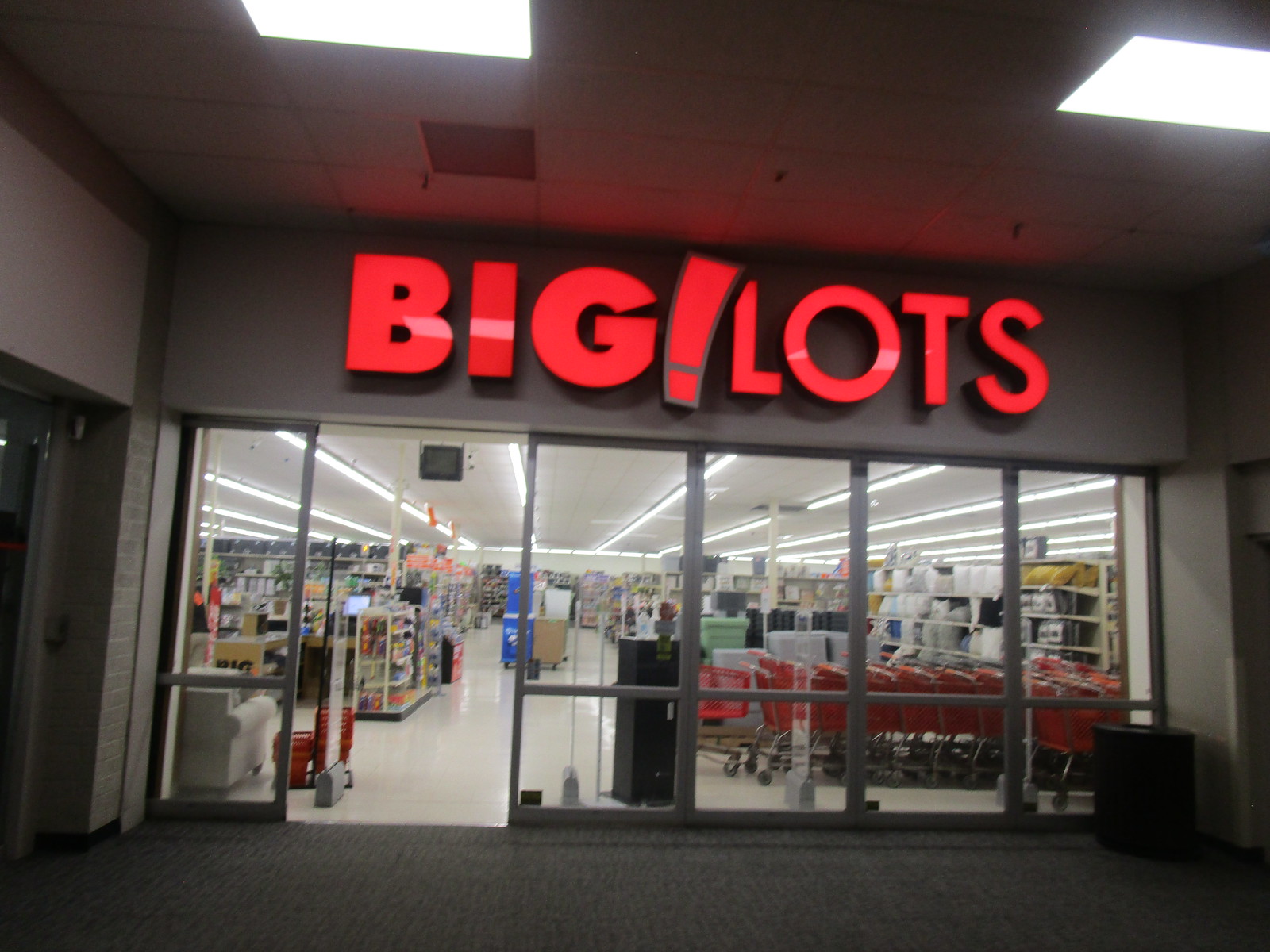This is a detailed, nighttime photograph of the exterior entrance to a Big Lots store, captured from the parking lot. The bright red illuminated letters spell "Big Lots" above the entrance, complete with the signature large exclamation point in the middle. The sliding glass door is open, revealing the interior of the store. Inside, you can see a row of orangish-red shopping carts lined up just past the doorway, and a stack of red plastic shopping baskets near a white upholstered armchair positioned with its back to the entry. The store features a black-and-white tiled floor and fluorescent lighting in a tiled ceiling. Various items for sale are visible, including trash cans, laundry baskets, knickknacks, and furniture, such as a white couch on the left. To the right, some pillows are stacked, while other aisles filled with merchandise extend deeper into the store.